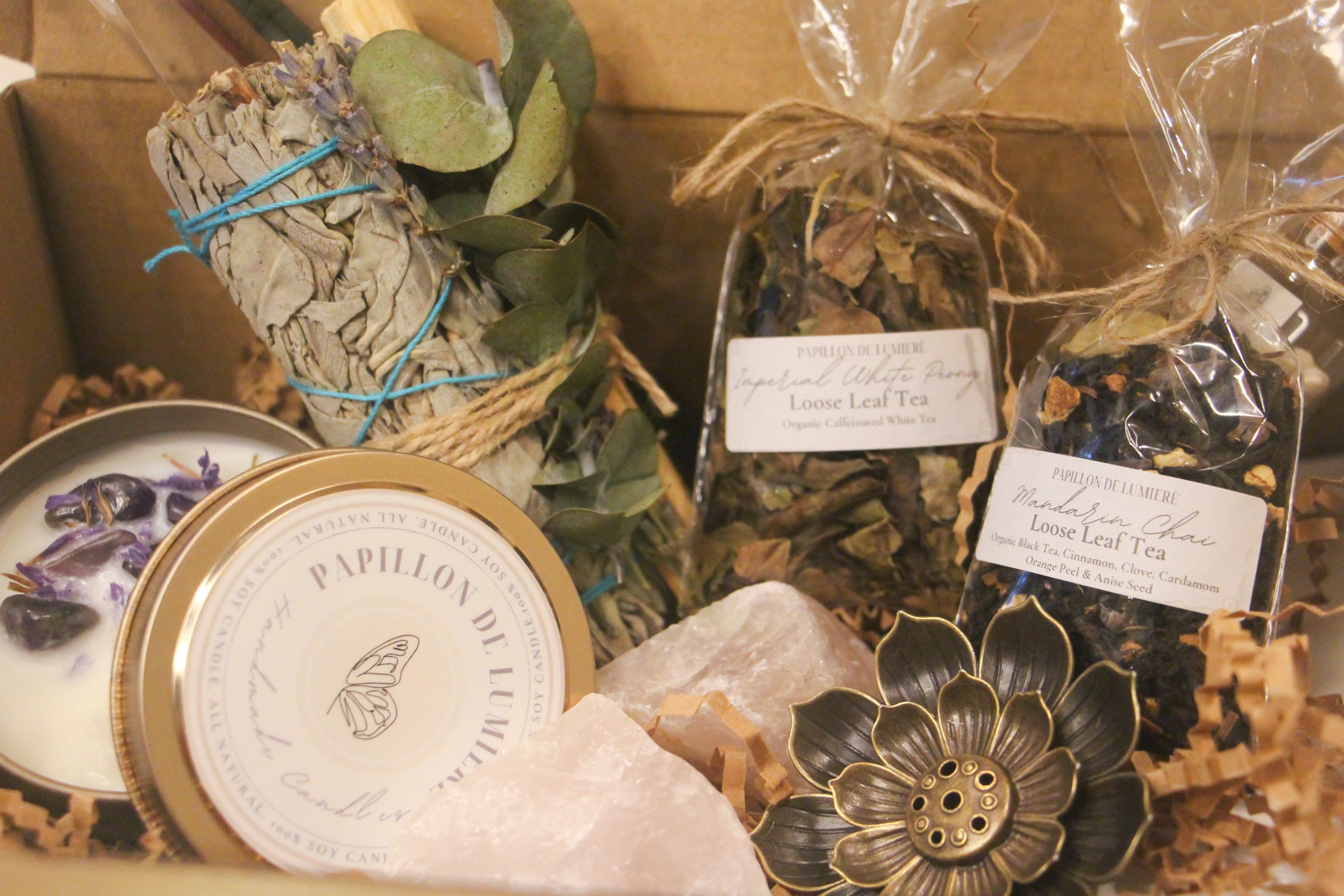This photograph presents a close-up view of a thoughtfully arranged gift basket within a thick, brown corrugated cardboard box. Dominating the lower left-hand corner is an open, milky tin containing what appears to be lavender leaves or flowers, possibly part of a soap or balm product, with its lid labeled "Papillon de Luminare" lying nearby. This tin is slightly obscured by two pieces of rose quartz. Adjacent to this setup is a large, metal flower emblem, lending a decorative touch to the arrangement.

In the background, several bundles of sage smudge sticks, each tied with blue string, are neatly placed. Accompanying these are two distinct bags of loose leaf tea: one labeled "Papillon de Luminare" and the other "Mandarin Chai." 

Additionally, there is a mention of a candle visible within the basket, its top removed to reveal a surface embedded with flowers, suggesting a fragrant, decorative element. The image evokes a sense of natural, soothing aromas, underlined by the inclusion of potpourri, wrapped in leaf bundles and sticks. Overall, the neatly-packed items suggest a curated selection of artisanal products, each contributing to the aesthetic and sensory appeal of the gift basket.